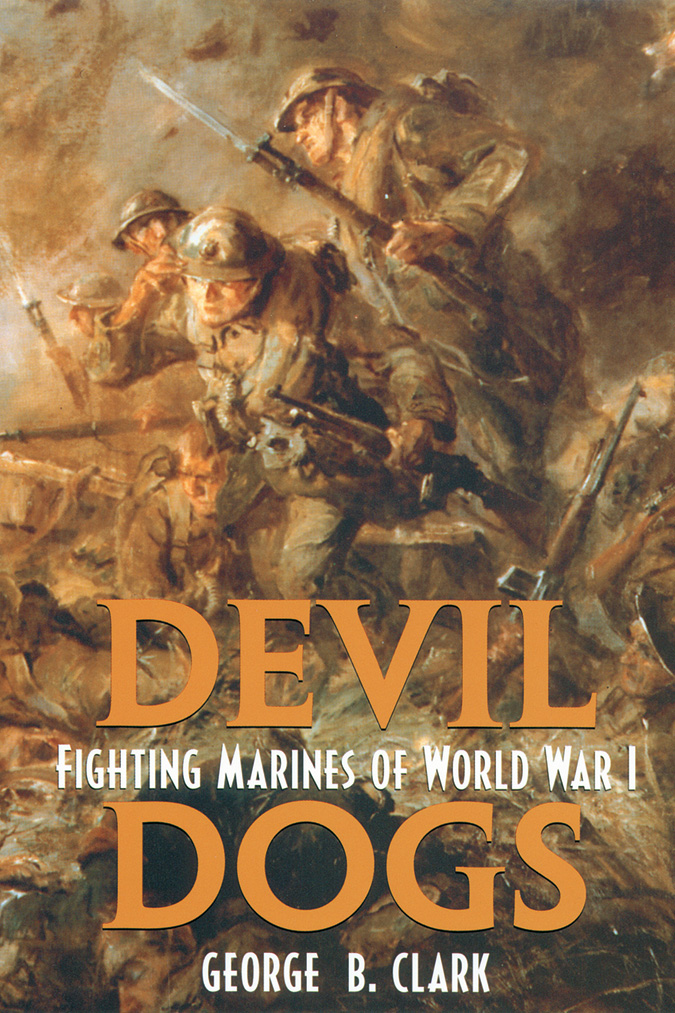The image is a detailed and impressionistic cover of a book titled "Devil Dogs: Fighting Marines of World War I" by George B. Clark. Dominated by neutral tones of brown, dark yellow, and rust, the illustration conveys a sense of chaos and urgency typical of wartime scenes. The foreground features three soldiers in army uniforms and helmets – two wielding bayonets and another with a rifle – all seemingly in motion as if running into danger. The background is a tumultuous mix of brown and brownish-pink, evoking a sky filled with dust and conflict. The soldiers appear to be in trenches or a bunker, under fire, with one possibly injured. The title, "DEVIL DOGS", is prominently displayed in large, orange rust-colored letters, with "Fighting Marines of World War I" in smaller white capitals beneath it, and the author's name, George B. Clark, at the bottom, also in white capitals. This vivid illustration effectively sets the tone for the historical content within, focusing on the bravery and turmoil of Marines during World War I.